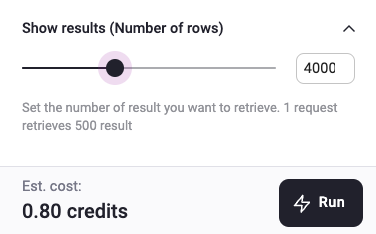The image depicts a user interface panel designed for managing and retrieving data results. At the top, there is a line of text that reads "Show Results (Number of Rows)" with "Close" in parentheses, indicating the ability to specify and display a certain number of data rows. Below this, a black line with a small black circle, surrounded by a light purple shading, acts as a graphical separator.

Next, there's a text box pre-filled with the number "4,000," which represents the number of results the user wants to retrieve. A small, black caret is located next to this input field, allowing the user to adjust the number of results.

Text below the input field states, "One request retrieves 500 results" and "Estimated cost: 0.80 credits." The estimated cost is highlighted in grey to signify its informational purpose. A horizontal grey line separates these sections, maintaining visual clarity and organization.

To the bottom right of the panel, a black button labeled "Run" in white text is prominently displayed, featuring a lightning bolt icon, suggesting the execution of the data retrieval process.

Overall, the panel's design is minimalist, using primarily black and white colors, except for the subtle touch of light purple around the black circle, and there are no indications of which website this interface belongs to.